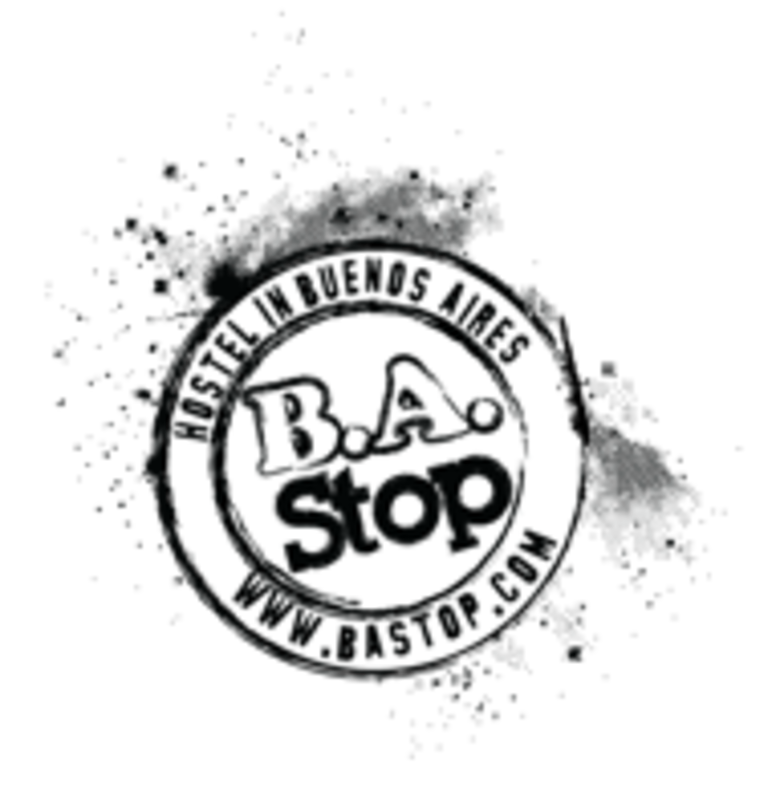This image displays a somewhat pixelated and blurry logo resembling a circular passport stamp typically found in a passport. The logo features a double border with the text "Hostel in Buenos Aires" along the upper perimeter and the website "www.bastop.com" along the bottom. At the center, in larger text, it reads "B.A." and just below it "Stop." The entire design is monochromatic, using black text on a white background. Surrounding the circle, there are artistic ink smudges and splatters, contributing to a stamped, textured look. The absence of additional objects or people emphasizes the focus on the logo itself.